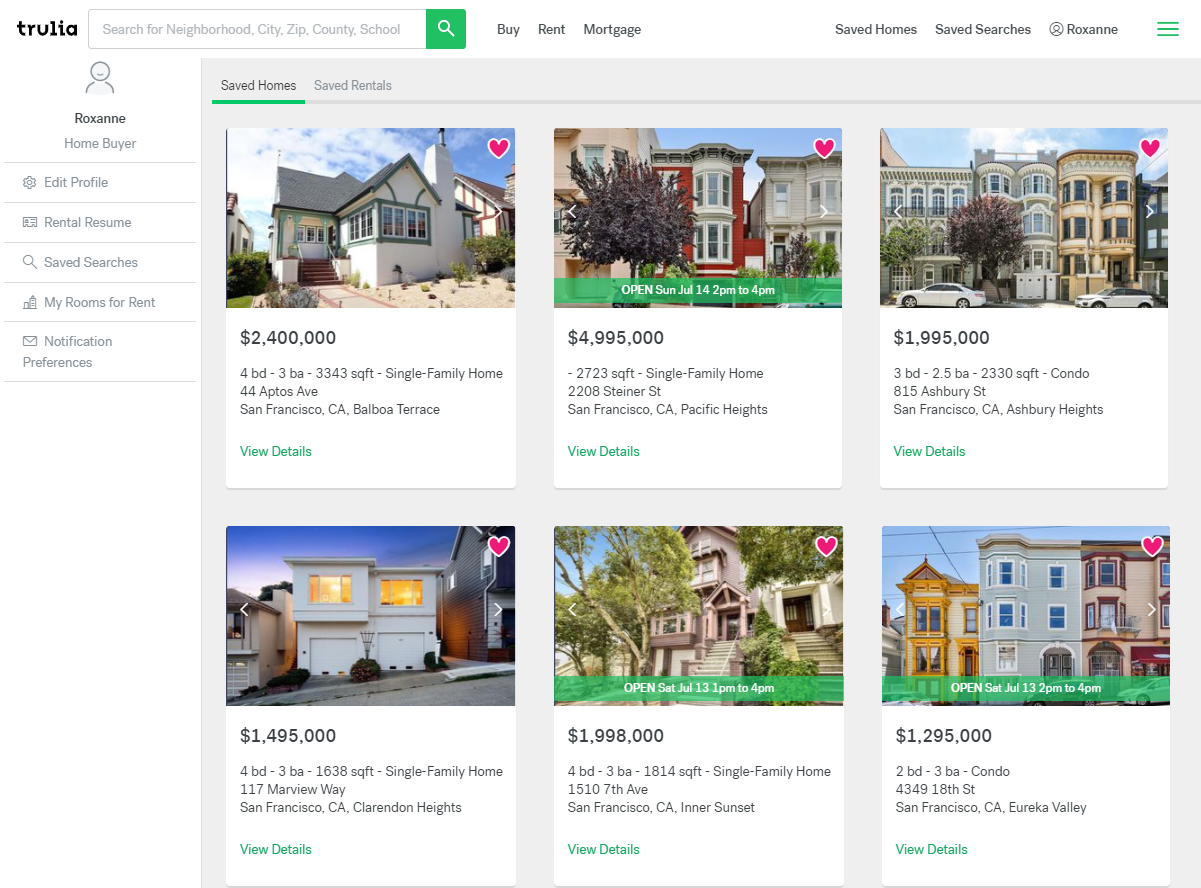The image displays a webpage from Trulia. At the top, there is a search field with placeholders for searching by neighborhood, city, zip code, county, or school. Various navigation options are outlined, including "Buy," "Rent," "Mortgage," "Saved Homes," "Saved Searches," "Homebuyer," "Edit Profile," "Rental Resume," "Saved Rentals," and "Notification Preferences."

On the right side of the page, a list of homes with their respective values is shown. These homes, all located in California, are listed as follows:
- The first property is valued at $2.4 million.
- The second property is priced at $4,995,000.
- The third property is listed at $1,995,000.
- The fourth home has a value of $1,495,000.
- The fifth property is priced at $1,998,000.
- The sixth home is valued at $1,295,000.

To the left of the page, there are quick access links labeled "Edit Profile," "Rental Resume," "My Rooms for Rent," and "Notification Preferences."